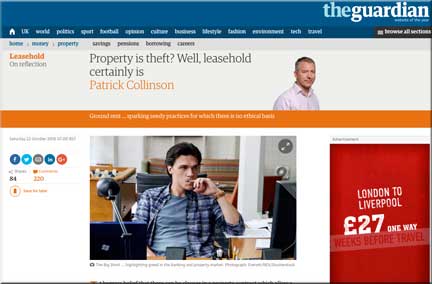The image displays a webpage from "The Guardian" website. At the top, it prominently features a navigation bar with links to various sections, including UK, World, Politics, Sports, Culture, Lifestyle, Tech, Travel, and Savings. The main headline on this page reads: "Property is Theft: Well, Leasehold Certainly Is," authored by Patrick Collinson. The page discusses issues related to leasehold. On the left side of the webpage, there are social media icons for sharing the article on Facebook, Twitter, LinkedIn, and Google Plus. At the bottom right corner, there's a highlighted advertisement promoting a travel deal: "London to Liverpool, £27 One Way."